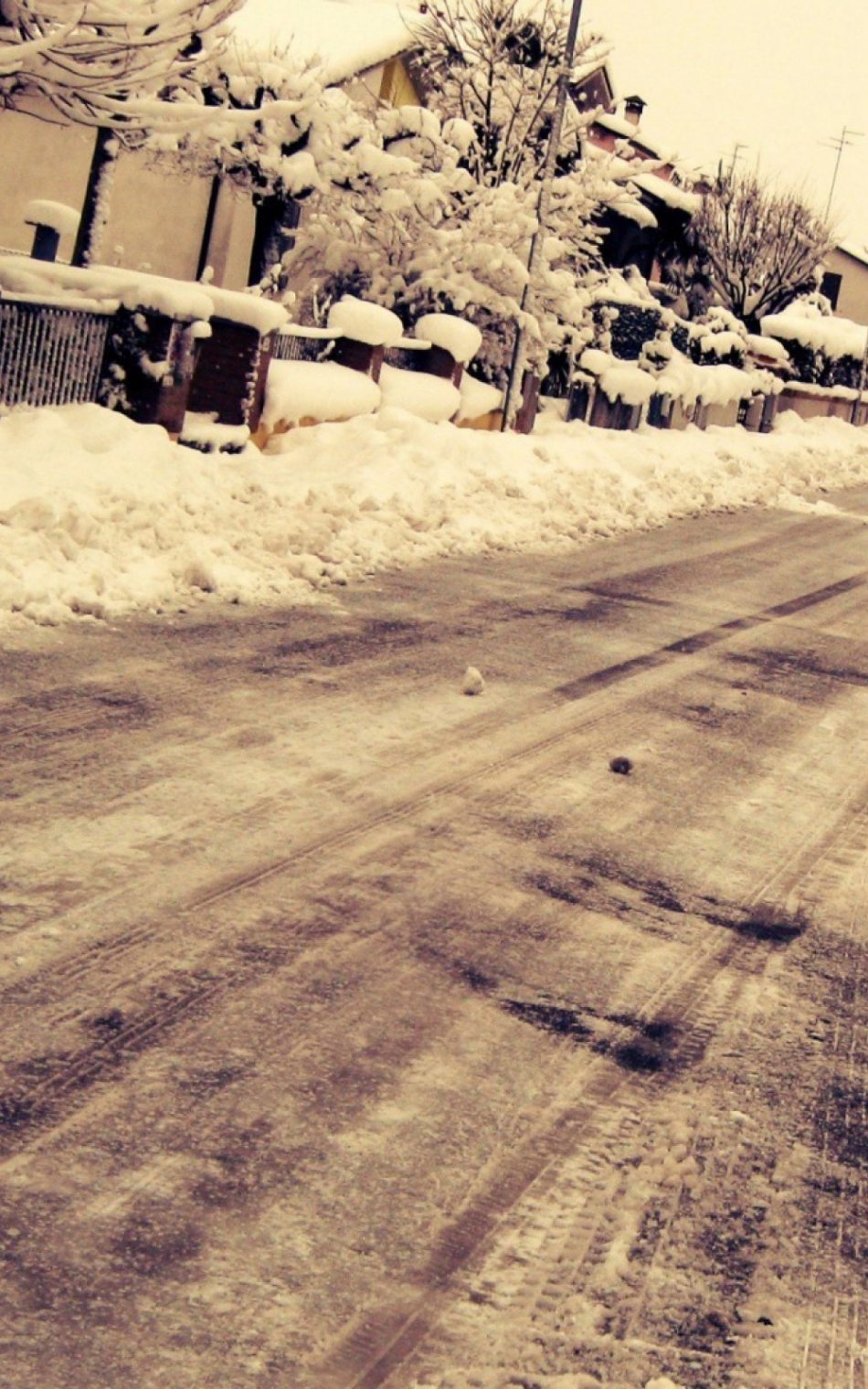This photograph, reminiscent of a sepia or old black-and-white image with a yellowish tint, captures a suburban street in winter. The main focus is the road, prominently positioned at the lower part of the image, displaying faint tire tracks from cars. Although the street itself has been recently plowed, showing only a thin layer of snow, snow is heavily piled up along the sides. 

On the left side of the road, the snow forms substantial mounds, partially concealing rubbish bins lined up along the street. Above these bins are house fronts or possibly a low-rise condo complex, characterized by triangular rooftops and chimneys. Utility poles and light posts rise above the scene, adding to the vintage suburban feel. 

The upper left section of the image features individual houses fenced off by structures with thick, snow-covered stone or brick columns. Bare trees with branches weighed down by thick layers of snow stand between the houses and the road, adding a stark, wintry beauty to the scene. The overall effect is a picturesque, almost timeless depiction of a quiet residential street blanketed in winter’s embrace.